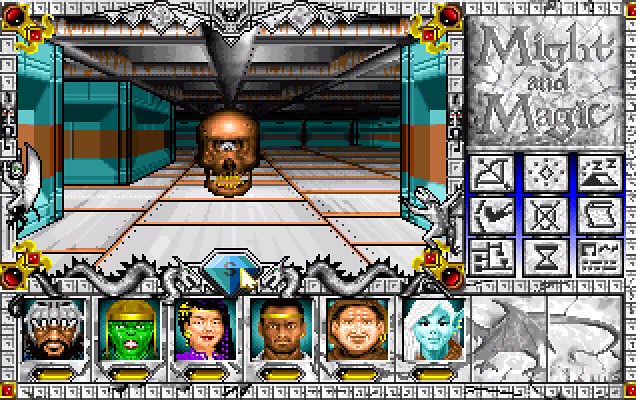This image is a detailed screenshot from the late 90s PC game "Might and Magic." Dominating the screen is the main game interface, showcasing an interior of a dungeon with light blue walls featuring brown stripes and recesses, which create a coffered ceiling effect. The focal point is a floating red skull with yellow teeth. In the background, more blue walls can be seen, forming a solid block-like structure. Above, in the top right corner, is the title "Might and Magic" in a gray box.

Below the main screen is a lineup of six character avatars: from left to right, they include a light blue elf with white hair, a monkey-like figure with a gold earring, a black man with a gold headband, a female in a purple outfit, a green alien-like figure with a metal hat, and another black man with a skull hat. To the left of these characters are multiple selectable icons featuring various items such as an hourglass, a crossbow, a tent, and more, likely representative of different gameplay actions or statuses.